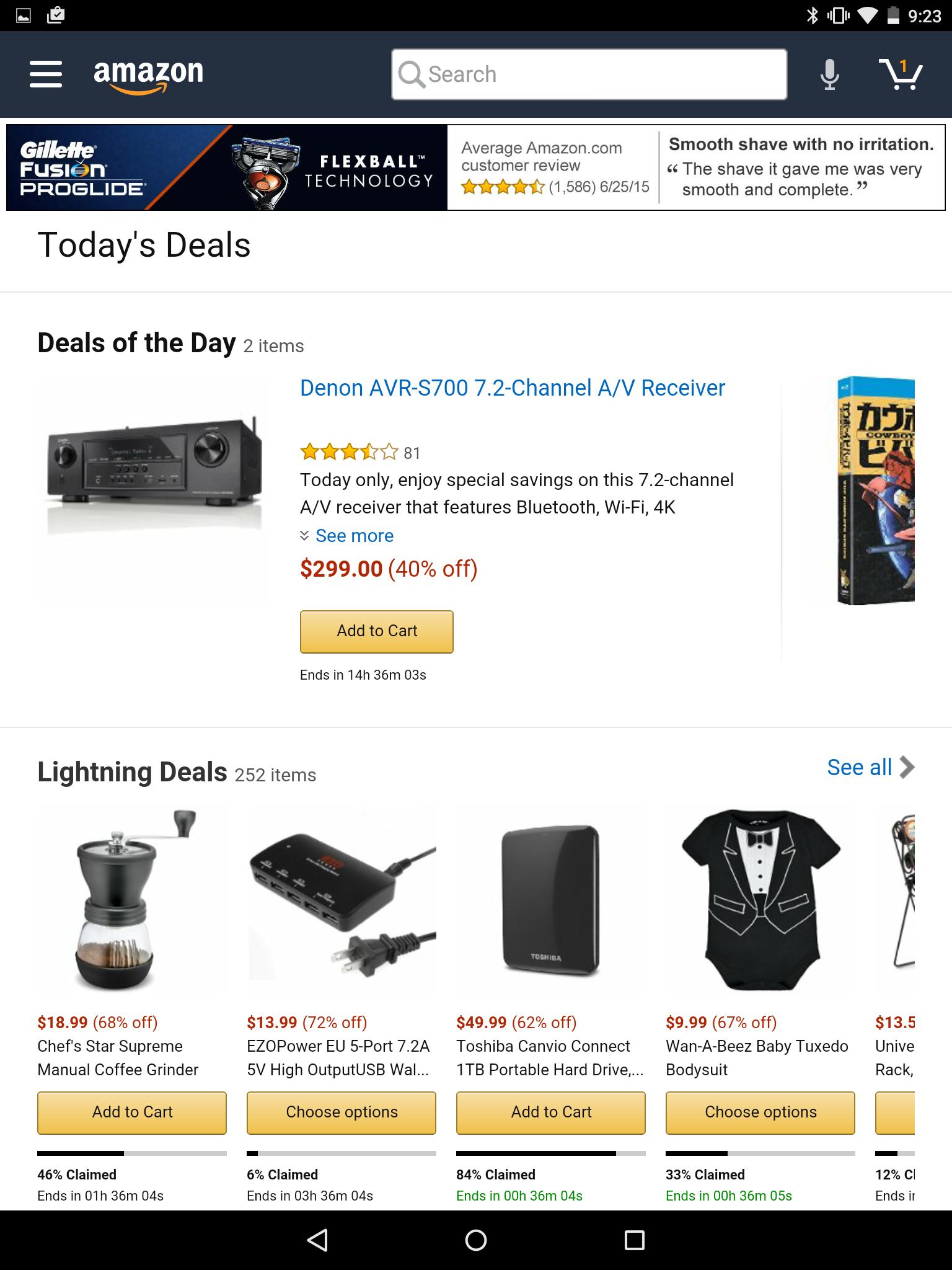A detailed description of the screenshot from the Amazon website displayed on a cell phone:

---

The screenshot captures a view of Amazon’s website on a mobile phone. At the very top, a black banner displays standard smartphone interface elements including cellular reception, a Bluetooth icon, and the time "9:23."

Directly below this, a dark gray banner stretches across with several key Amazon branding and functional elements. On the left, three horizontal white lines indicate the main menu. Next to it is the Amazon logo, consisting of the text "Amazon" with an arrow that curves upward to form a smile. Following this, a search bar features a white magnifying glass icon, and a white microphone icon for voice search. On the far right, a white shopping cart icon with a yellow badge reveals there is one item in the cart.

Beneath the Amazon banner is an advertisement for the Gillette Fusion ProGlide razor. The ad includes a product image, the average customer review rating of just over four stars from 1,586 reviews, and a feedback comment dated June 25, 2015, that reads: "Smooth with no irritation. The shave it gave me was very smooth and complete."

Following the ad, there is a section for "Today's Deal" showcasing the "Deal of the Day," which is the Denon AVR-S700 7.2 Channel A-V Receiver. To the left is an image of the AV receiver with text highlighting its Bluetooth features. The product possesses slightly over three-star reviews. The accompanying text states: "Today only, enjoy special savings on this 7.2 channel AV receiver that features Bluetooth." On the right edge, a partial image of another item is visible but cut off.

Further down, 252 items are listed as lightning deals, though only four are visible in the screenshot:

1. **Chefstar Supreme Manual Coffee Grinder**: Listed for $18.99, which is 60% off, with an "Add to Cart" button beneath it.
2. **EZO Power EU547.2A 5V High Output USB Wall Charger**: Price and discount not entirely visible but has a "Choose Options" button underneath.
3. **Choshiba Kenevo Connect 1TB Portable Hard Drive**: Priced at $49.99, a 62% discount, with an "Add to Cart" button below it.
4. **Juan Abez Baby Tuxedo Bodysuit**: Includes a "Choose Options" button, though price details are not completely visible.

The clean and organized layout combines functionality and appealing promotions, typical of Amazon's user-friendly interface.